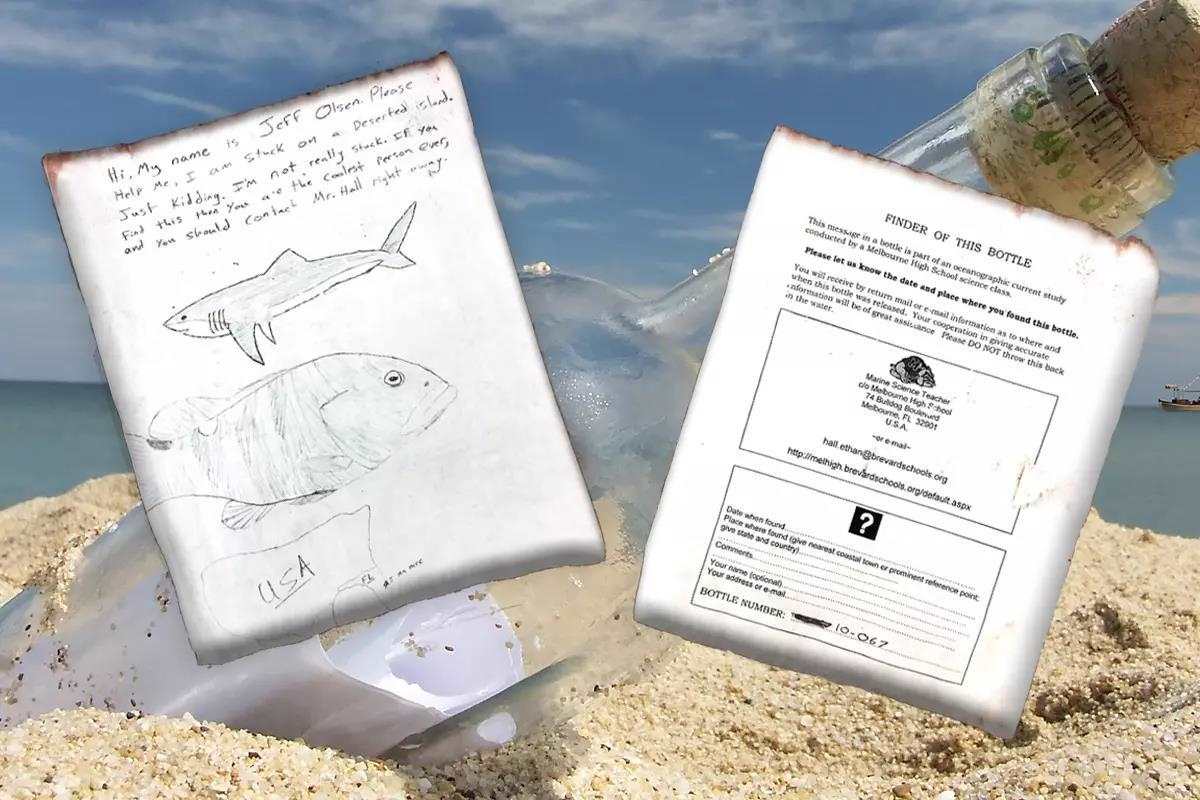A vibrant, full-color outdoor photograph captures the whimsical scene of a clear glass bottle lying partially buried in the golden sand, sealed with a cork and containing a rolled-up piece of paper. The image takes place on a mostly sunny day, utilizing natural light to create a bright and cheerful atmosphere. In the background, the sparkling ocean stretches out beneath a blue sky dotted with a few soft clouds. Superimposed onto the image are two photoshopped white pieces of paper. The one on the left features playful hand-drawn illustrations of a shark and a fish, along with a lighthearted message that reads: "Hi, my name is Jeff Olson. Please help me. I am stuck on a deserted island. Just kidding. I'm not really stuck. If you find this, then you are the coolest person ever and you should contact Mr. Hall right away." The paper on the right seems more formal, providing detailed instructions on what to do if the bottle is found, potentially indicating that the entire setup is part of a creative class project.